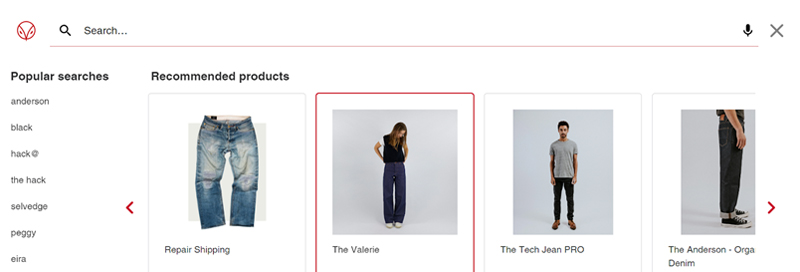This screenshot captures a segment of an online clothing shopping interface. At the top, there's a search bar flanked by two icons: on the left, a red circle resembling an owl's face with a downward-pointing triangle and small dots representing eyes; on the right, a microphone icon and an 'X' to close the search bar. 

The left-hand navigation panel lists "Popular Searches," including terms: Anderson, Black, Hack (with an indiscernible icon), The Hack, Selvage, Peggy, and Eira. 

To the right of this panel lies the "Recommended Products" section, showcasing four items. The first product is titled "Repair Shipping" featuring an image of light blue jeans with white accents on the thigh area. The second product, "The Valerie," highlighted with a red outline, depicts a woman dressed in black pants, a black vest, and a white t-shirt. The third item, "Tech Jean Pro," presents a man clad in jeans, brown shoes, and a gray shirt. The final product, "Anderson Orga Denim," displays a lower body shot of a person wearing dark jeans and Converse shoes, extending from the waist down and showing part of their arm.